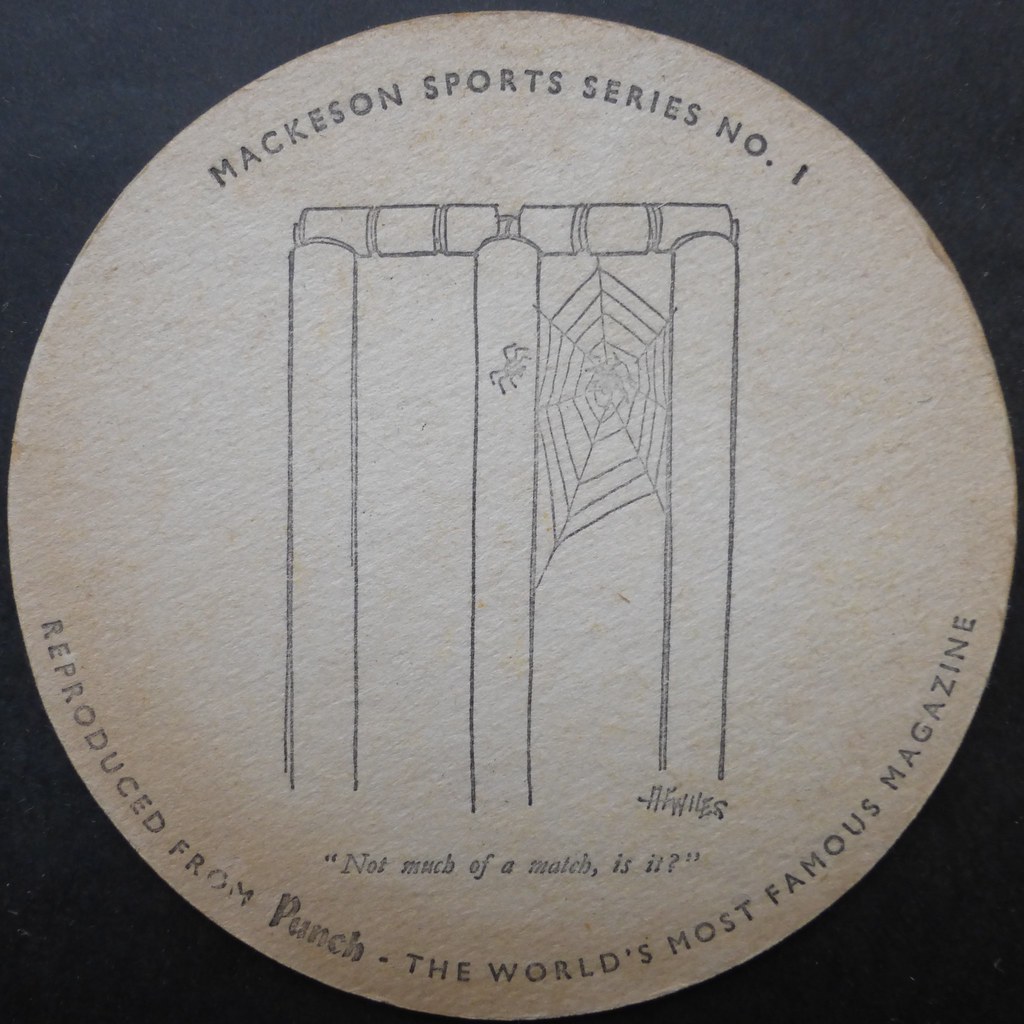This photo depicts a large, brown coaster or button resting on a black background. The coaster appears to be made from a material resembling cardboard or thin-edged wood. It features a faded black inscription at the top that reads "Maxon Sports Series Number One" and at the bottom, "Reproduced from Punch, the world's most famous magazine." Just above the bottom text, there is a quote saying, "Not much of a match, is it?"

Central to the coaster's design is an intricate drawing. The illustration seems to depict large playground bars or wooden dowels, but could also be interpreted as two books stacked on top of each other. The artwork showcases a spider sitting on a central bar, while to the right, a larger web holds another spider in its midst, potentially engaged in a silent standoff. Below this drawing, there is a signature that appears to read "A.F. Wiles," though it is slightly obscured and difficult to decipher. The spiders and the detailed web scene bring life to this aged and artistic coaster, making it a captivating piece.